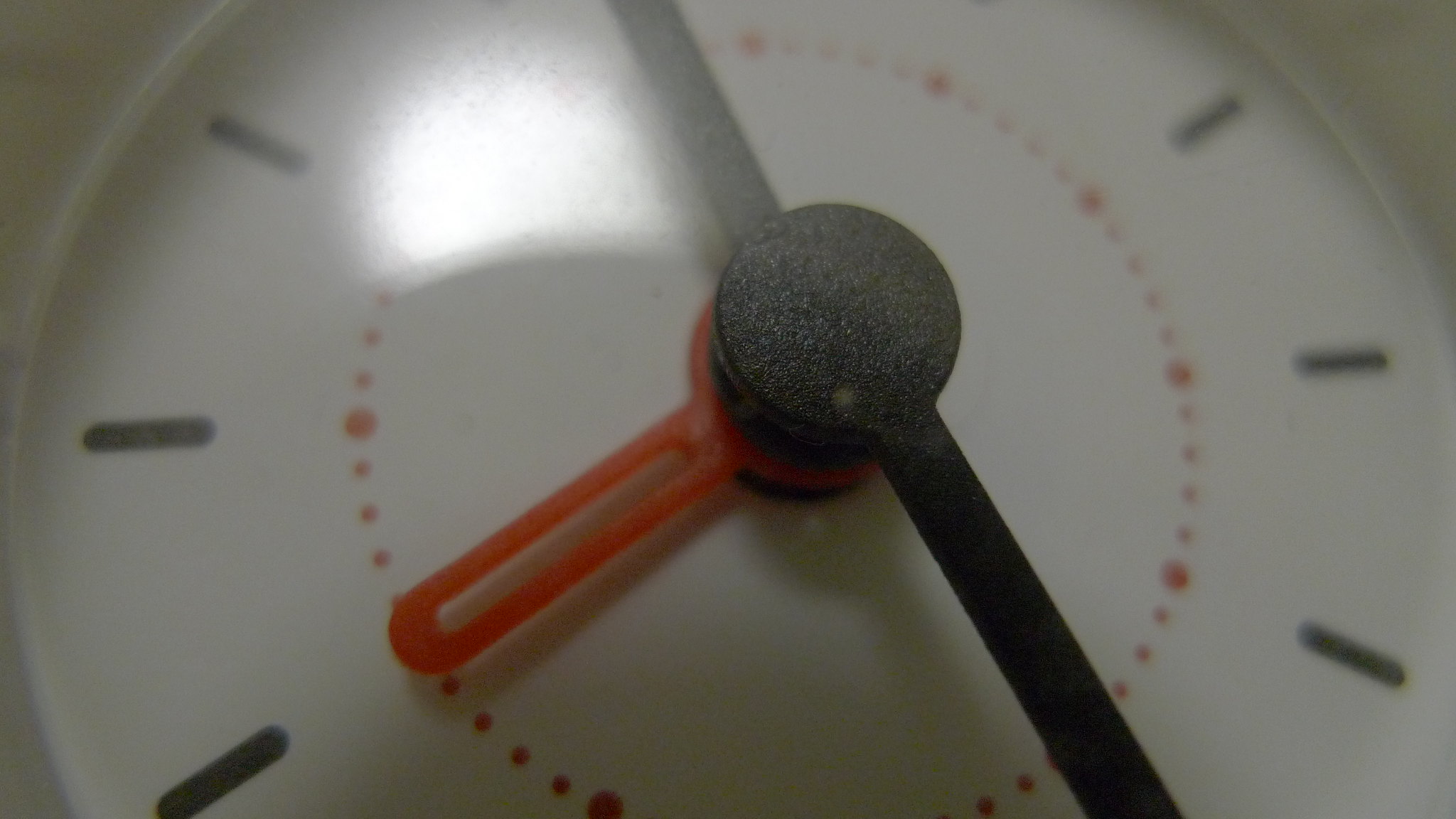This horizontally-oriented macro photograph captures a partially visible analog clock, conveying a sense of time's fleeting nature through its slight blur. Dominating the center of the image, the clock's hour and minute hands stretch diagonally from the upper middle section towards the lower right. A red second hand, distinctive with its curved shape and central hole, adds a dynamic element, casting soft shadows across the clock face. Surrounding the clock's inner dial are small red dots, while simple black lines mark the outer perimeter, providing a minimalist yet functional design. A subtle reflection graces the clock's protective glass or plastic cover near the red second hand, adding depth to this detailed portrayal of time.